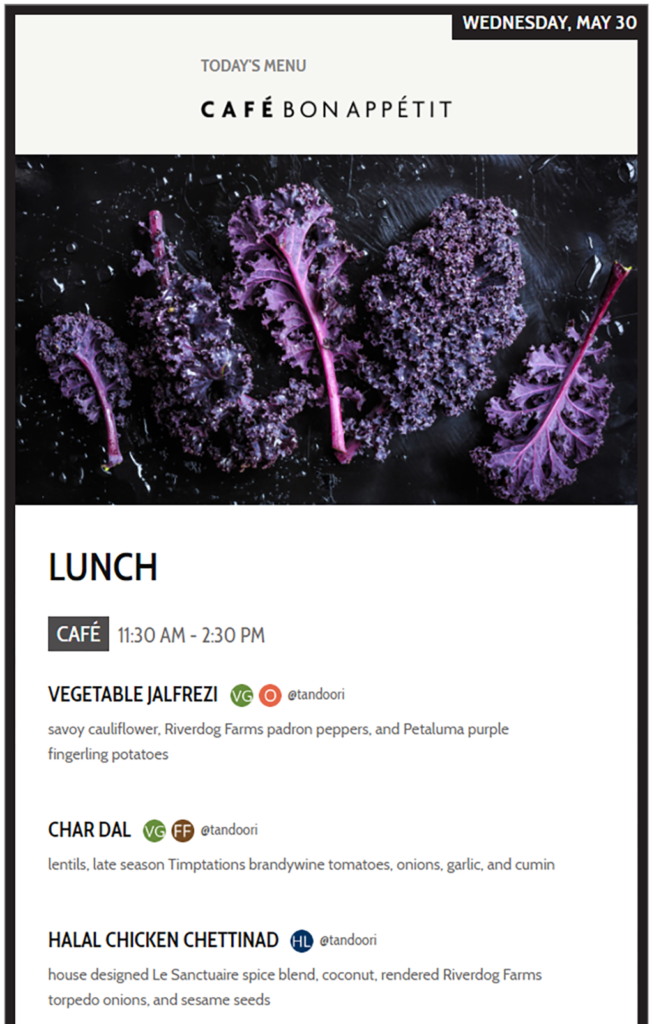The image is a digital representation of a restaurant menu from "Cafe Bon Appetit." At the very top of the webpage is the name of the establishment, prominently displayed. Directly below the cafe's name is a high-resolution, vividly colored image showcasing five pieces of lettuce. The striking brightness of the lettuce suggests that the image has been digitally enhanced, which might raise questions about the authenticity of the presentation.

Beneath the enhanced image, the menu section is clearly marked as "Lunch," listing the available offerings. The listed items include "Vegetable Jalfrezi," "Chardale," and "Halal Chicken Cheddanad." Additionally, the operational hours of the cafe are noted in this section.

The overall design of the menu is modern and sleek, with no distracting background elements, focusing solely on the vivid visual and the menu items. Despite the possible over-enhancement of the lettuce image, the presentation is professional and high-quality, aiming to entice potential customers with its colorful and clean layout.